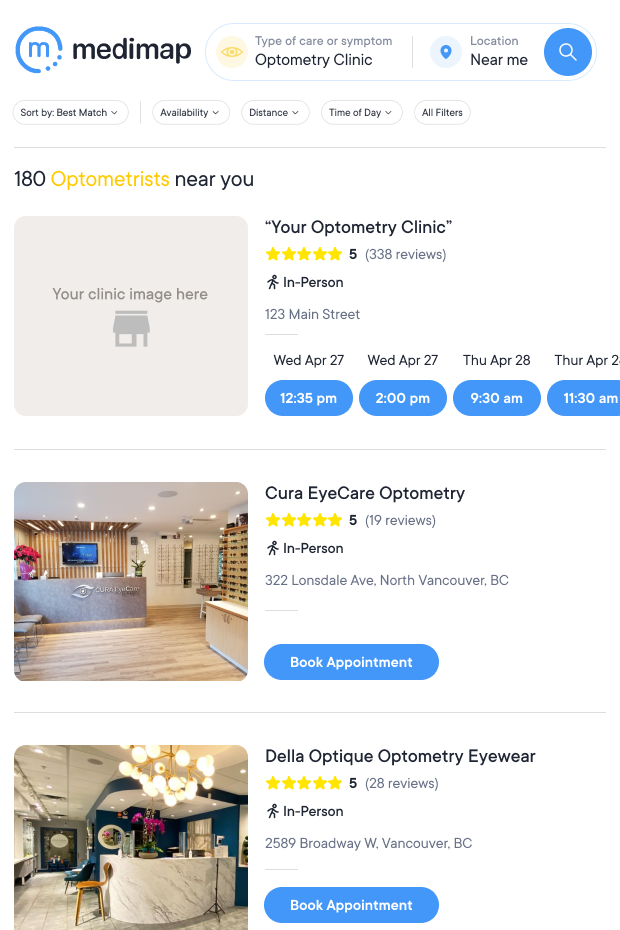In the upper left corner of the image, there is a media map and a distinctive logo. The logo features a blue circle partially composed of three dots, with a lowercase letter "m" centered inside. To the right of this logo, there is a search field labeled "Type of Care or Symptom," in which "Optometry Clinic" is typed out. Another search field labeled "Location" is adjacent, containing the text "near me." 

Next to these search fields is a circular search icon resembling a magnifying glass. Below the search fields, there are various dropdown menus for refining the search results: "Sort Best By," "Best Match," "Availability," "Distance," "Time of Day," and "All Filters."

A horizontal line separates these menus from the search results below. The search results indicate there are 180 optometrists near your location. The first result lists your optometry clinic, rated five stars based on 338 reviews. The clinic offers in-person visits at 123 Main Street and has availability on the following dates:

- Wednesday, April 27th at 12:35 p.m.
- Wednesday, April 27th at 2:00 p.m.
- Thursday, April 28th at 9:30 a.m.
- Thursday, April 28th at 11:30 a.m.

All the available appointment times are displayed in blue buttons with white font.